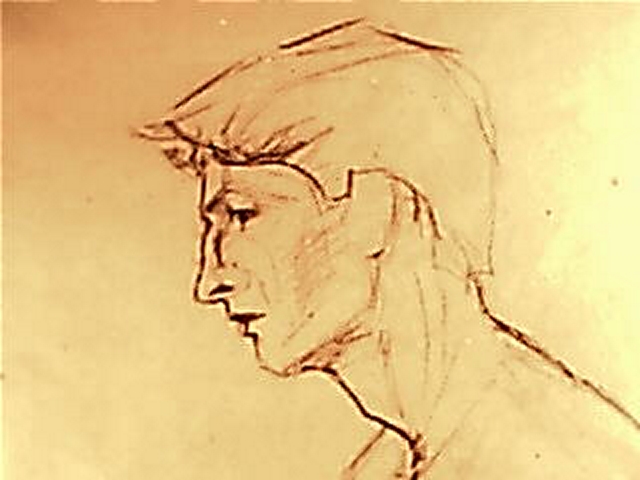This image is a hand-drawn sketch of a young man on a multi-colored paper background that transitions from light greens and taupes to a darker taupe, with hints of peach and ivory. The paper has a yellowish-orange tint, possibly due to the lighting or the image quality. The drawing itself is a profile view of the man, who appears to be looking slightly downwards to the left, giving him a pensive or sad expression. 

The man's hair is brushed forward and sticks up above his forehead without resting on it, cut short around his ears, and it appears uncolored, possibly suggesting a blonde hue. His eyebrows are dark, almost black, matching his black eyes and eyelashes. He has a prominently shaped Roman nose, angular and well-defined. His mouth is closed, and his strong chin and long neck, with an Adam's apple visible, extend down to his bare shoulder, indicating he might not be wearing a shirt. The drawing uses thick black outlines and lacks detailed shading, emphasizing the basic contours of his face and head.